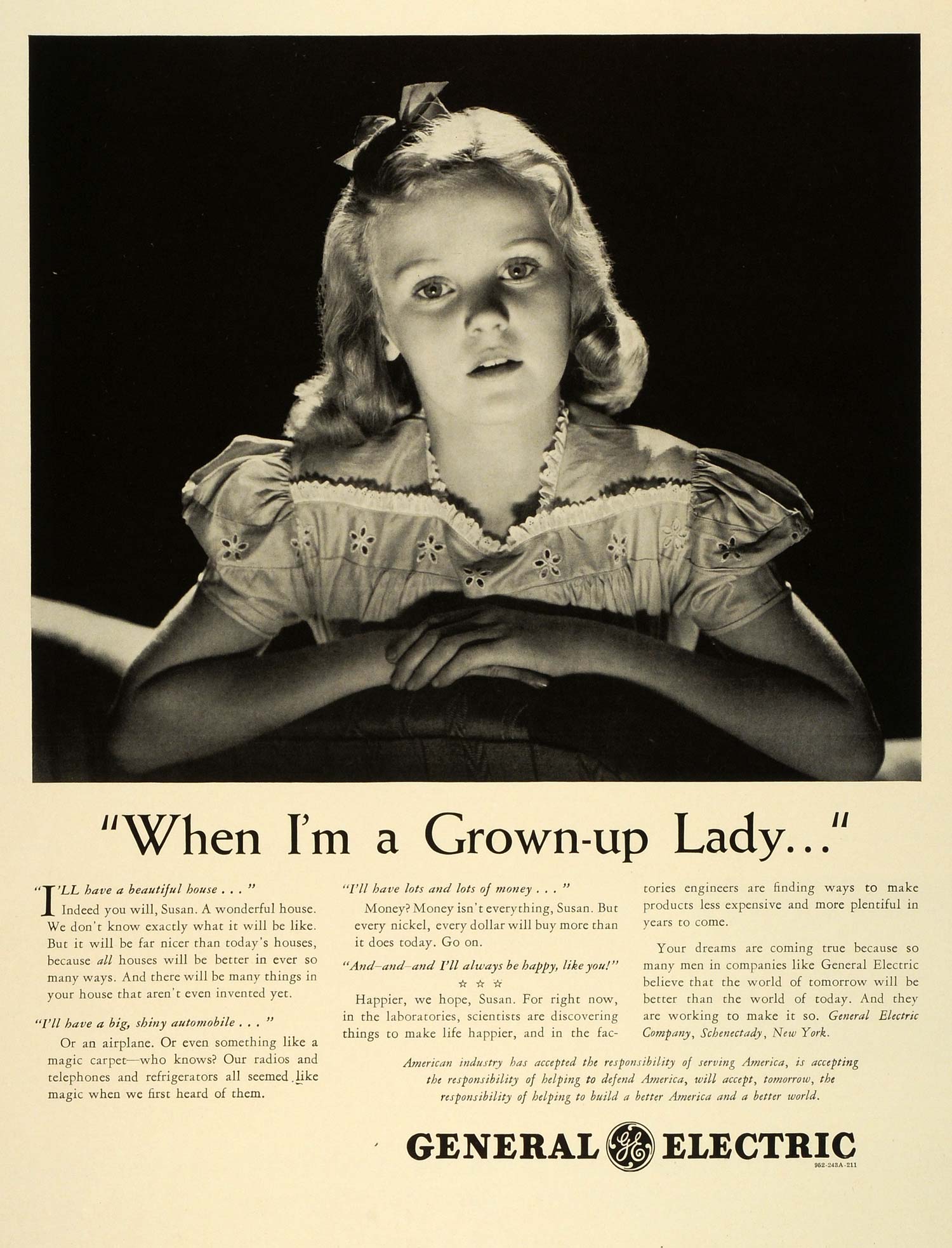The image is an advertisement for General Electric, depicting a yellowed magazine page with a large black-and-white photograph that occupies more than half of the space. The photograph captures a young, blonde girl, likely around 8 to 10 years old. She has shoulder-length, curled hair adorned with a bow on the left side. The child is dressed in an older-style frilly dress with puffy sleeves, and she poses by leaning forward on a chair with her arms folded. Her expression is slightly docile, with her head slightly tilted and her gaze directed straight at the camera.

Beneath the image, the title "When I'm a Grown-Up Lady" is prominently displayed in large serif font and quotations. Below this title, there's a column of smaller text organized in a narrative that reflects the girl's dreams about her future. Lines from the text read, "I'll have a beautiful house. Indeed, you will, Susan, a wonderful house...all houses will be better in ever so many ways...I'll have a big, shiny automobile or an airplane or even something like a magic carpet...I'll have lots and lots of money...I'll always be happy like you...Happier, we hope, Susan..."

The text emphasizes the vision of a better future, stating that engineers and scientists from General Electric are working to make new inventions and more affordable, abundant products. The ad concludes with the company's name and location, "General Electric Company, Schenectady, New York," and a message conveying the company's responsibility towards building a better America and world. The General Electric logo is prominently featured at the bottom of the advertisement.